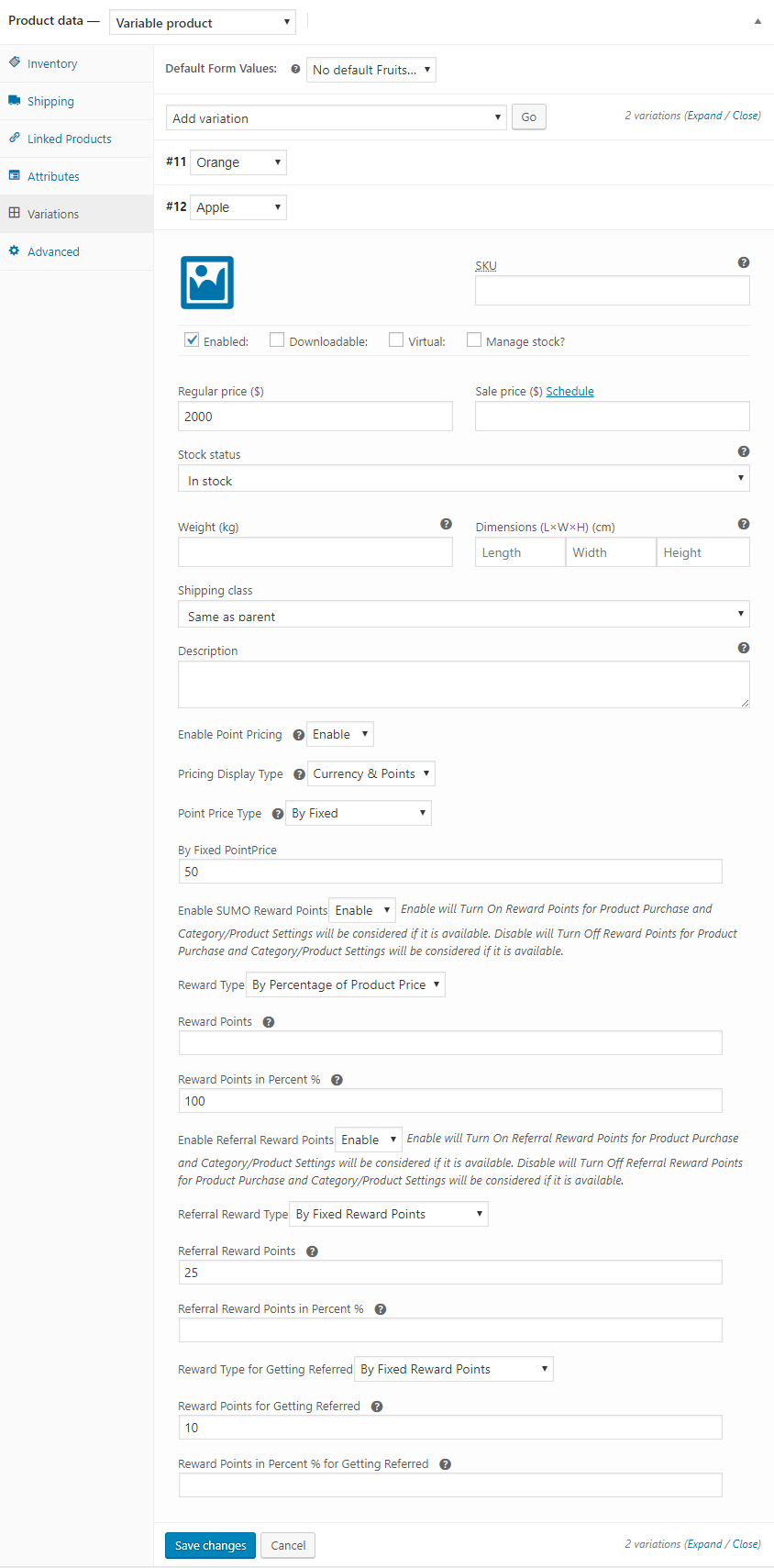This image depicts a detailed configuration form on the administrative backend of an e-commerce website, likely aimed at configuring product variations. 

### Overview
- **Tabs**: Positioned at the top left are two prominent tabs:
  - "Product Data" (active in black)
  - "Variable Product" (also in black)
  
- **Sidebar Menu**: Running vertically down the left side against a slightly off-white background is a blue menu with the following options:
  - Inventory
  - Shipping
  - Linked Products
  - Attributes
  - Variations (active tab, in black)
  - Advanced
  - Each menu item features a small blue icon to its left.

### Variation Form
The right-hand side hosts the main form, beginning with two secondary tabs:
  - "Default Form Values"
  - "No Default Fruits"

Beneath these tabs is a gray text entry bar labeled "Add Variation" with a "Go" button on the right.

### Variation Entries
The form includes multiple text entry fields and dropdowns:
  - Two primary entries: 
    - **11 (Orange)**
    - **12 (Apple)**
  - These entries feature gray down arrows on their right side, indicating dropdowns.

### SKU and Stock Management
- **SKU Field**: On the far right, labeled "SKU" with a gray information bubble at the top right.
- **Enabled**: A checkbox, ticked in blue, indicates that the variation is enabled.
- **Additional Labels** (not checked):
  - Downloadable
  - Virtual
  - Manage Stock?
- **Price Fields**:
  - Regular Price: "2000"
  - Sale Price: Adjacent to it, there's a blue "Schedule" hyperlink.
- **Stock Status**: Indicates "In Stock" with an adjacent weight entry window left blank.
- **Dimensions**: Fields for length, width, and height are present.

### Shipping and Description
- **Shipping Class**: Displays "Same as Parent" with a dropdown arrow.
- **Description**: A large white text box labeled "Description" with a gray information bubble in the top right corner.

### Enable and Pricing Options
- Three rows of selectable lists:
  - "Enable Point Pricing": Checked.
  - "Pricing Display Type": "Currency and Points".
  - "Point Price Type": "Fixed".

### Reward Points
- **Enable SLIMO Reward Points**: Contains a descriptive paragraph, followed by:
  - "Reward Type": "Percentage of Product Price".
  - A blank reward points entry window.
  - Reward points percentage: 100%.
  - "Enable Referral Reward Points": Enabled, with an accompanying paragraph.
  - "Referral Reward Points": 25.
  - "Referral Reward Points Percent": Empty.
  - Reward points for getting referred: 10.
  - Percentage for getting referred: Empty.

### Action Buttons
- **Save Changes**: Blue button with white text, positioned on the left.
- **Cancel**: White button with black text, located on the right.

This extensive form provides a comprehensive interface for managing product variations, including inventory, pricing, shipping, and reward points functionalities. The user-centric design ensures each input field and option is clearly labeled and organized for ease of use.